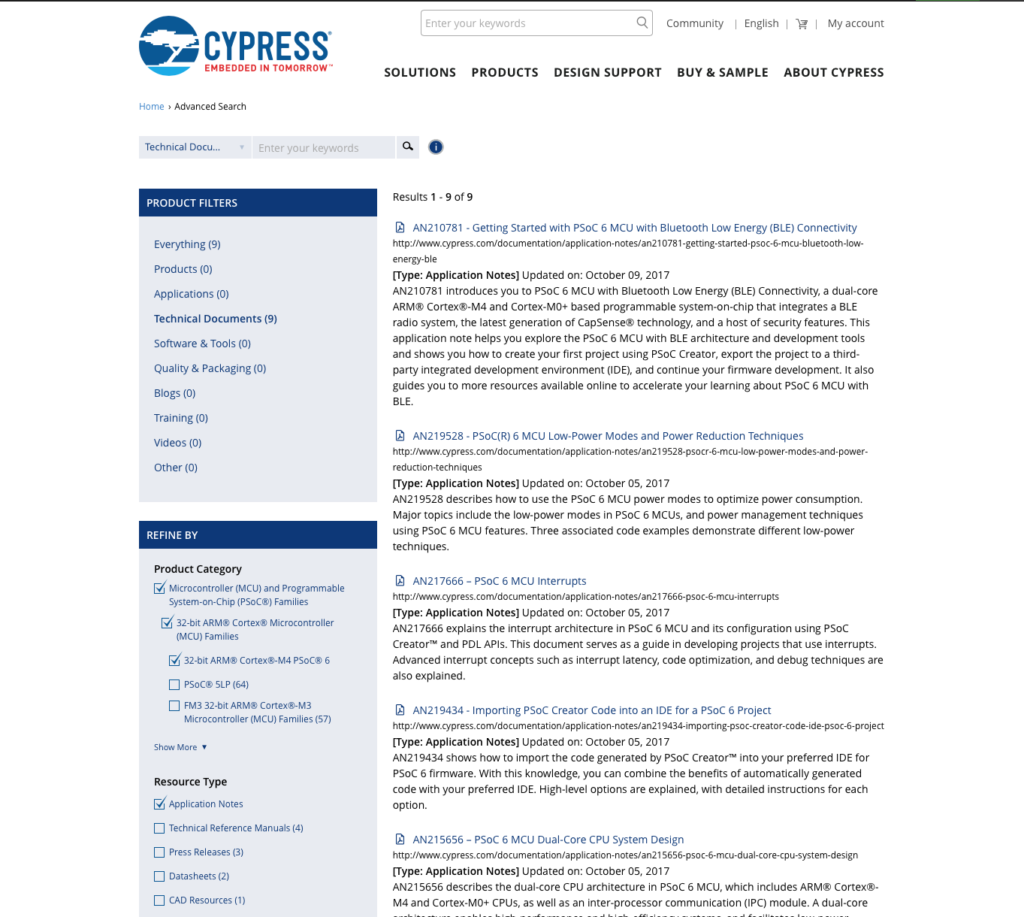In this image, we have a screenshot of a website associated with a company named "Cyprus," recognized by its tagline "Embedded in Tomorrow" and a circular emblem depicting a Cyprus tree. Positioned to the right of the logo is a search bar prompting users to "Enter your keywords," followed by navigation options including "Community," "English," a shopping cart icon, and "My Account." Beneath this header is a horizontal menu with clickable sections: "Solutions," "Products," "Design Support," "Buy and Sample," and "About Cyprus."

Continuing further down, there is a breadcrumb navigation indicating "Home" and an "Advanced Search" option, followed by another search bar with partially visible text "technical documents" and a magnifying glass icon. On the left side, a vertical sidebar lists various categories starting with "Product Filters" and encompasses "Everything," "Products," "Applications," "Technical Documents," "Software and Tools," "Quality and Packaging," "Blogs," "Training," "Videos," and "Other."

Below this list, another section labeled "Refined By" includes options with checked boxes such as "Product Category," "Microcontroller (MCU)," and "Programmable System on Chip (PSoC) Families." Further down are additional categories like "32-bit ARM Cortex Microcontroller (MCU) Families" and the "32-bit ARM Cortex M4 PSoC6."

To the right of this sidebar is a primary content area filled with text, primarily product descriptions and links. One highlighted example reads: "Type: Application Notes. Updated: October 9, 2017. AN210781 introduces you to PSoC6 MCU with Bluetooth Low Energy (BLE) connectivity, a dual-core ARM Cortex M4 and Cortex M0-based programmable system on chip that integrates with a BLE radio system, the latest generation of CapSense technology, and a host of security features," followed by further detailed information. The page appears to be heavily focused on technical specifications and product details related to microcontroller technology.